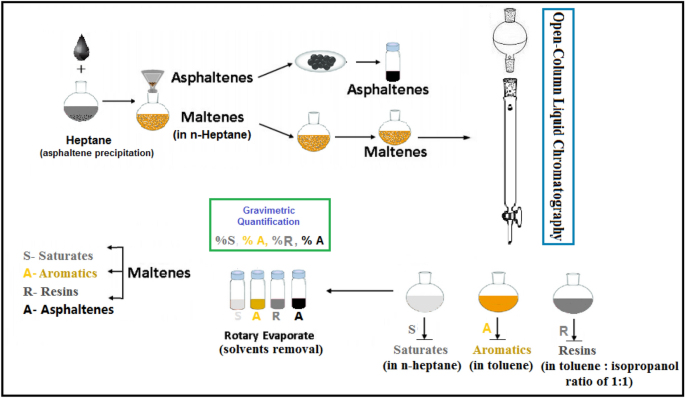The image is a detailed scientific diagram illustrating the process of open column liquid chromatography, prominently stated in a vertical light blue-outlined box to the right. The left side shows a droplet of gray liquid labeled as "heptane" next to a vial indicating "asphaltene precipitation." The diagram branches out to separate paths for "asphaltenes" and "maltenes," with arrows indicating their respective directions. Asphaltenes follow an upward arrow towards a circle filled with small black or gray particles and are labeled accordingly. Maltenes are directed downward, leading to a yellow vial marked "maltenes."

Further explanations below categorize maltenes as S (saturates), A (aromatics), R (resins), and A (asphaltenes), represented in a color-coded gravimetric quantification box: %S in gray, %A in yellow, %R in gray, and %A in black. Four small capped jars labeled S, A, R, and A indicate rotary evaporation for solvent removal. An arrow from the maltenes section points to three flasks on the right, colored gray, orange-yellow, and darker gray, detailing the solvents they contain: saturates in N-heptane, aromatics in toluene, and resins in a toluene-isopropanol mixture (1:1 ratio). This diagram effectively illustrates the step-by-step separation and identification process within open column liquid chromatography used in scientific analysis.